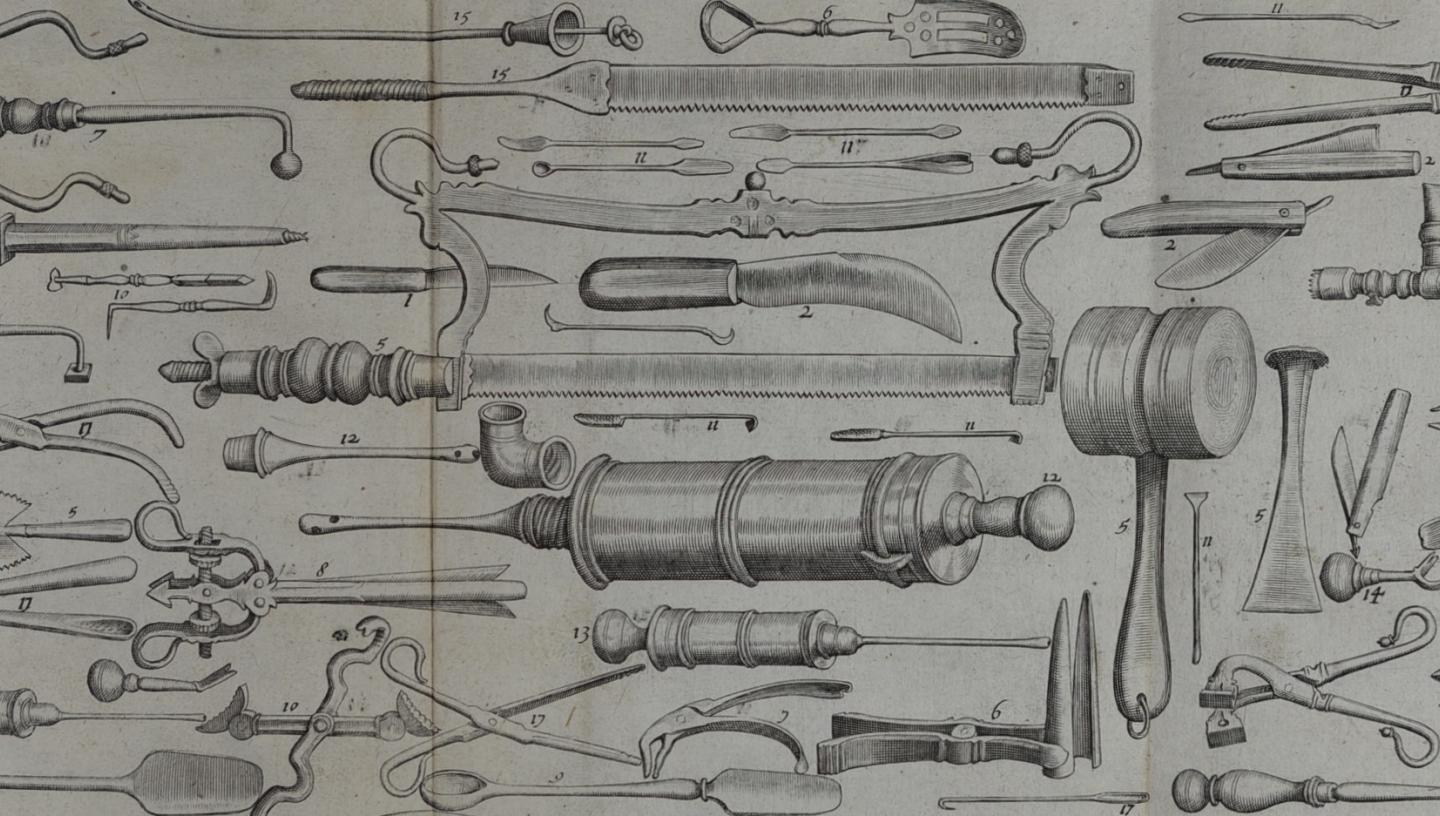The image depicts an old etching, intricately drawn in black ink on a grayish background. It features a comprehensive array of hand tools and parts, meticulously covering the entire canvas in a landscape orientation. Among the tools, one can identify a hand saw with a wooden handle, various types of knives including a curved knife, several kinds of pliers, and pocket watches. At the top, there’s another saw, while the center showcases a cylindrical object with a bellows and a handle. Scissors and clamps are also present, alongside other instruments like mallets, chisels, spatulas, and what resembles a sword or pick. Each item is labeled with numbers, though some numbers are repeated, such as the five seen on both a mallet and a chisel. Despite the absence of a legend to clarify the numbering, the image's detailed craftsmanship evokes a classical, almost historical, ambiance.